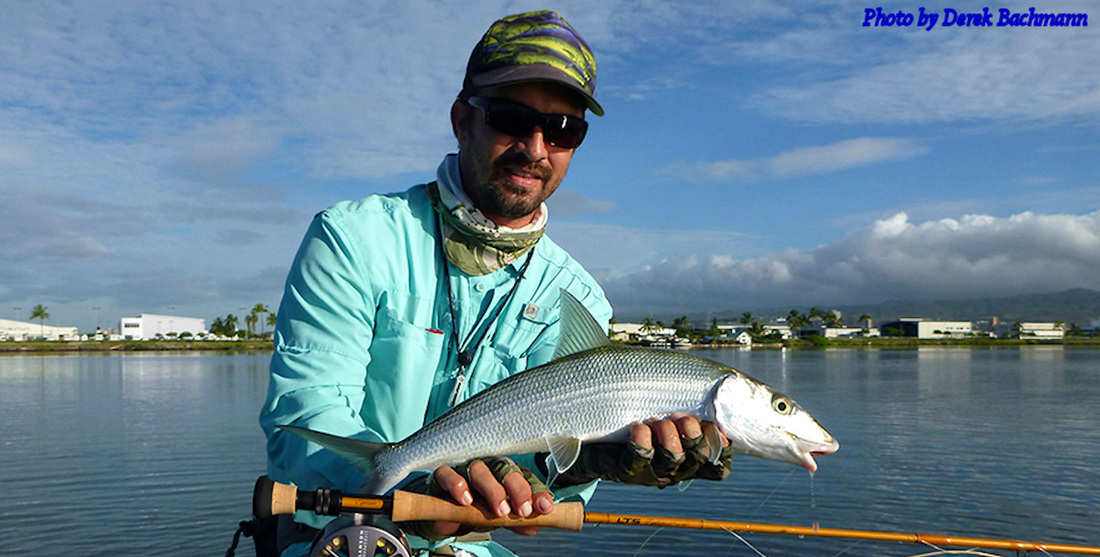This daytime photograph, taken by Derek Bachman, captures a serene outdoor scene by a calm body of water, possibly an ocean or a lake. The backdrop features a collection of white buildings and houses nestled along the shoreline, framed by abundant tropical palm trees. The sky above is a clear, brilliant blue, punctuated by heavy clouds on the bottom right-hand side. 

In the foreground, a man stands in the water, holding a two-foot-long fish he has just caught. He is dressed in a blue, long-sleeve shirt and protective hat adorned with images of fish, and wears black sunglasses. His fishing pole is in one hand, emphasizing the successful capture. The image has the text "Photo by Derek Bachman" placed in the top right corner.